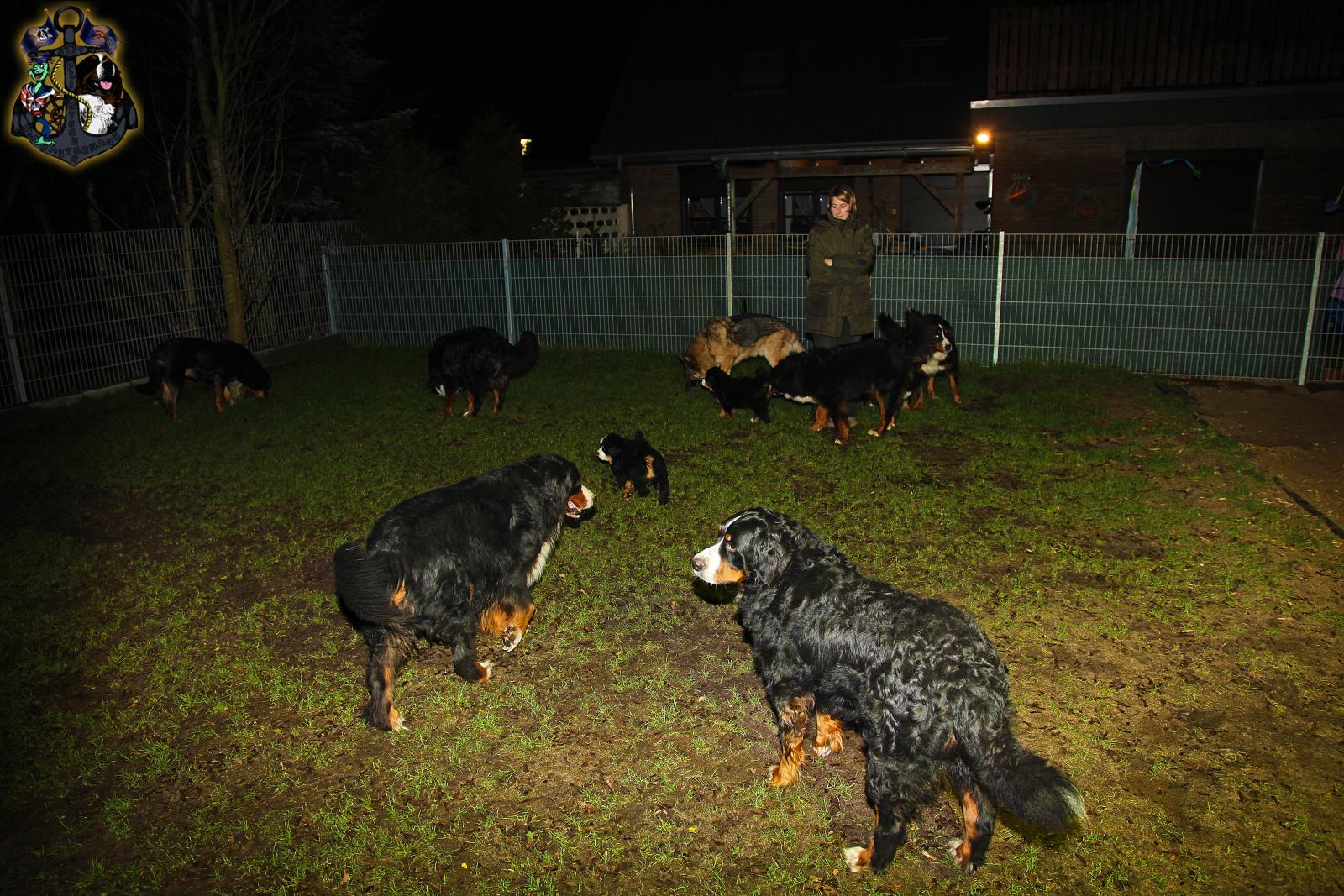In this color photograph taken at night in someone's fenced backyard, there is a gathering of nine dogs, mostly of a similar type, likely resembling Burmese Mountain Dogs, with black, shaggy coats, brown legs, white toes, and white and beige muzzles. Their lively, joyous demeanor is evident as they roam the grassy area, engaging in typical canine activities such as sniffing each other. Among them are a couple of smaller puppies. One notable outlier is a medium-sized dog with a tan coat and black saddle markings, possibly a German Shepherd. Standing watch over this scene is a woman with short blonde hair, wearing a long olive green winter coat. She stands near the entrance, surrounded by several of the dogs. In the background, a single-story house with a light on is visible next to an open garage door. In the upper left corner of the image, there is a distinct symbol resembling a gray anchor intertwined with a dog and possibly a snake, adding an enigmatic touch to the scene.